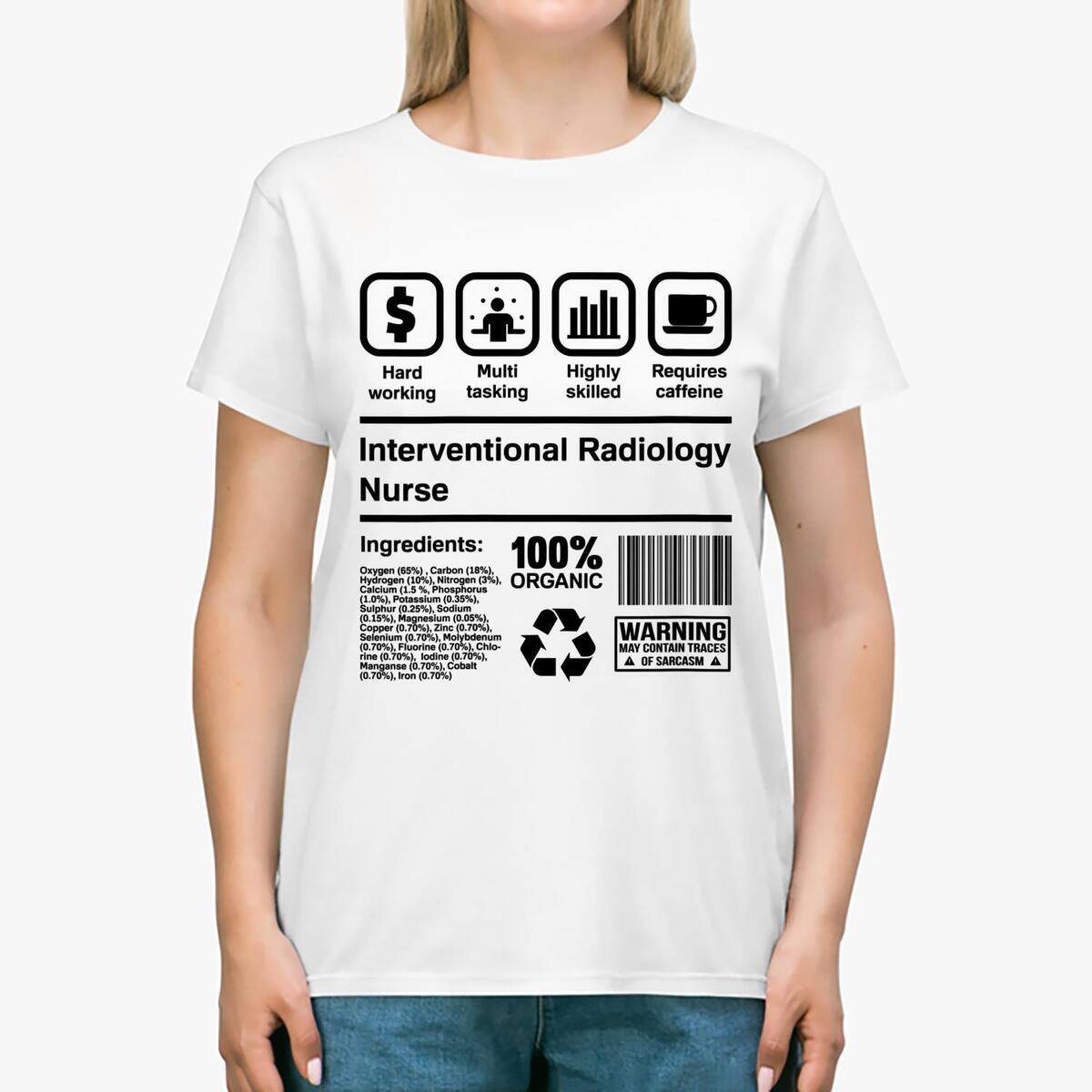The image features a woman with blonde hair modeling a custom white t-shirt with short sleeves. The t-shirt's design mimics a product label and includes various witty and informative text and symbols in black font. At the top of the shirt, it says "Interventional Radiology Nurse" and showcases iconography such as a dollar sign inside a cube labeled "Hard-working," a figure with connecting dots titled "Multitasking," a bar graph captioned "Highly Skilled," and a coffee mug with the text "Requires Caffeine" beneath it. Additionally, the shirt declares "100% Organic" and features a barcode at the bottom right. A humorous warning reads "May Contain Traces of Sarcasm." On the bottom left, the shirt lists its "ingredients" as elements like oxygen, carbon, hydrogen, nitrogen, calcium, and phosphorus, humorously reflecting the composition of a human being. The overall effect is a light-hearted, comedic representation of an interventional radiology nurse's dedication and multifaceted skills.